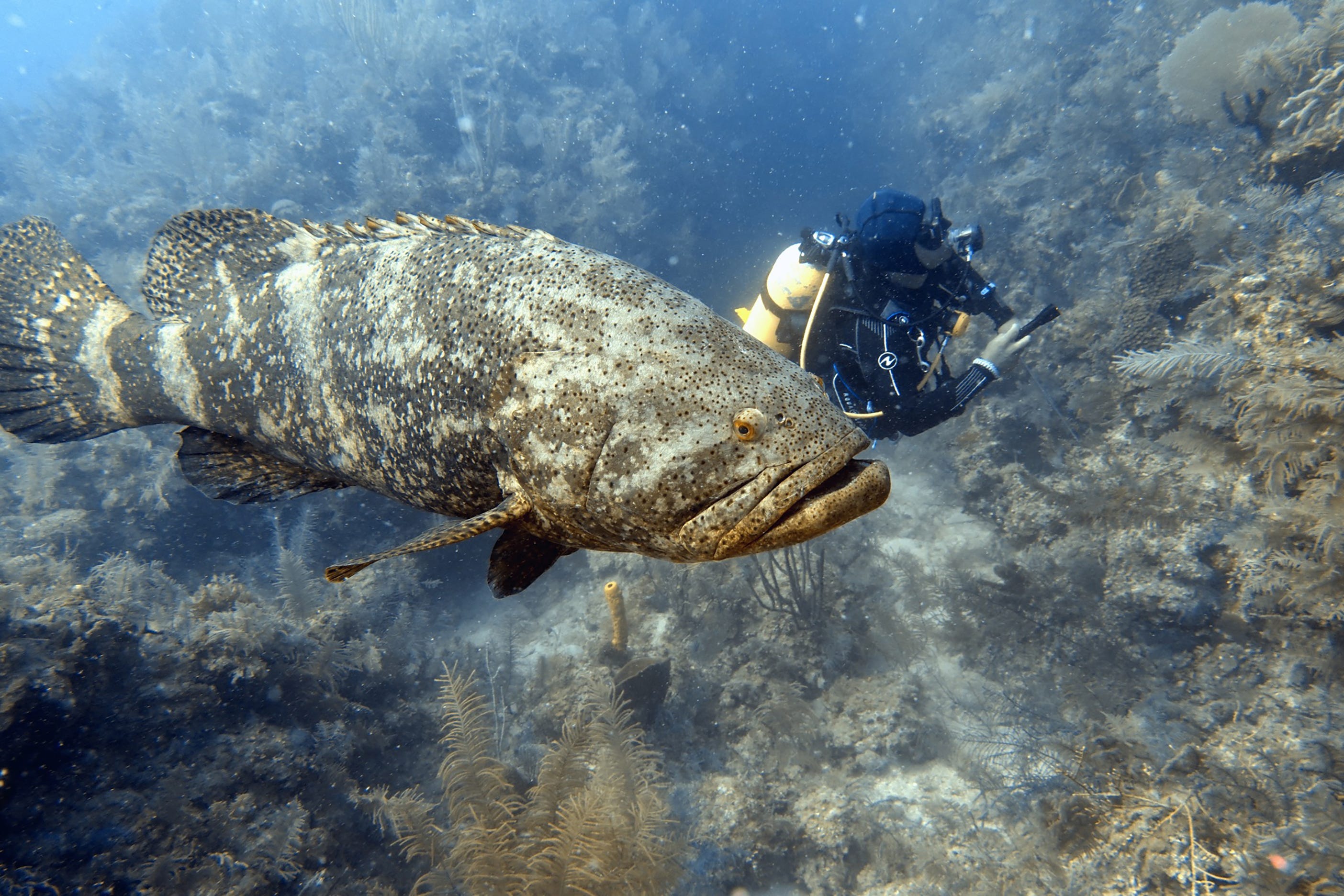The underwater photographic image captures a large grey fish, likely a grouper, swimming from left to right across the frame. Its tail fin reaches the left edge of the image, while its open mouth is positioned about two-thirds across the picture from left to right. The fish, adorned with white markings and dark scales, features an orange eyelid encircling a black eye. Two front fins are visible alongside its grey tail fin. Behind the fish is a scuba diver, clad in a black diving suit with a yellow oxygen tank. The diver, possibly holding a flashlight, has white gloves and a visible letter "N" or "Z" on their sleeve. Surrounding them is an ocean environment filled with predominantly grey underwater plants and some lighter green ones. The backdrop includes various reef and rock structures, with a notably dark area or hole behind the diver. The scene is illuminated naturally, resulting in a bright and clear image.